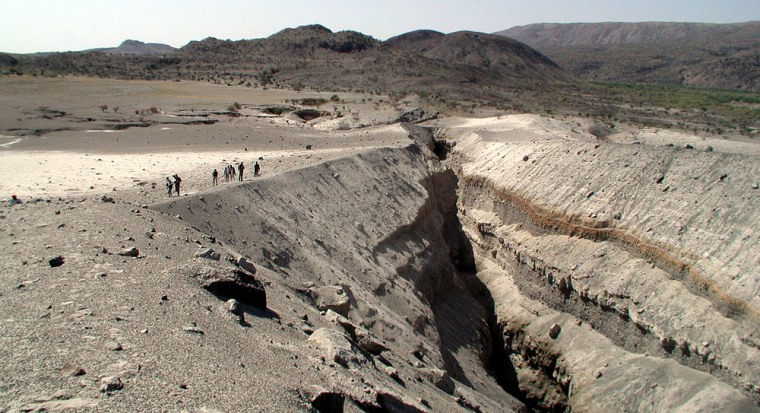This detailed image captures a striking desert landscape, dominated by an expansive and canyon-like fault line that cuts across the center of the photo. The foreground is teeming with details of rugged terrain characterized by layers of cracked, barren earth that fade from light tan to dark brown and orange hues, indicative of millennia of geological formations. Shadowy depths plunge into an almost pitch-black gorge, deepening the scene's dramatic effect. To the left, several individuals are visible, seemingly peering and walking along the edge of this chasm, suggesting a human scale to the vastness and depth of the fault line. Their presence hints at a possible exploration or touristic activity. In the background, one can observe gentle desert hills sparsely dotted with light greenery, accentuating the aridness of the location. The right side of the image is marked by a steep, imposing slope, emphasizing the formidable nature of this geological split. The starkness and seeming isolation evoke a sense of remoteness, underscoring the landscape’s stark beauty and suggesting a distant, undeveloped landmark.